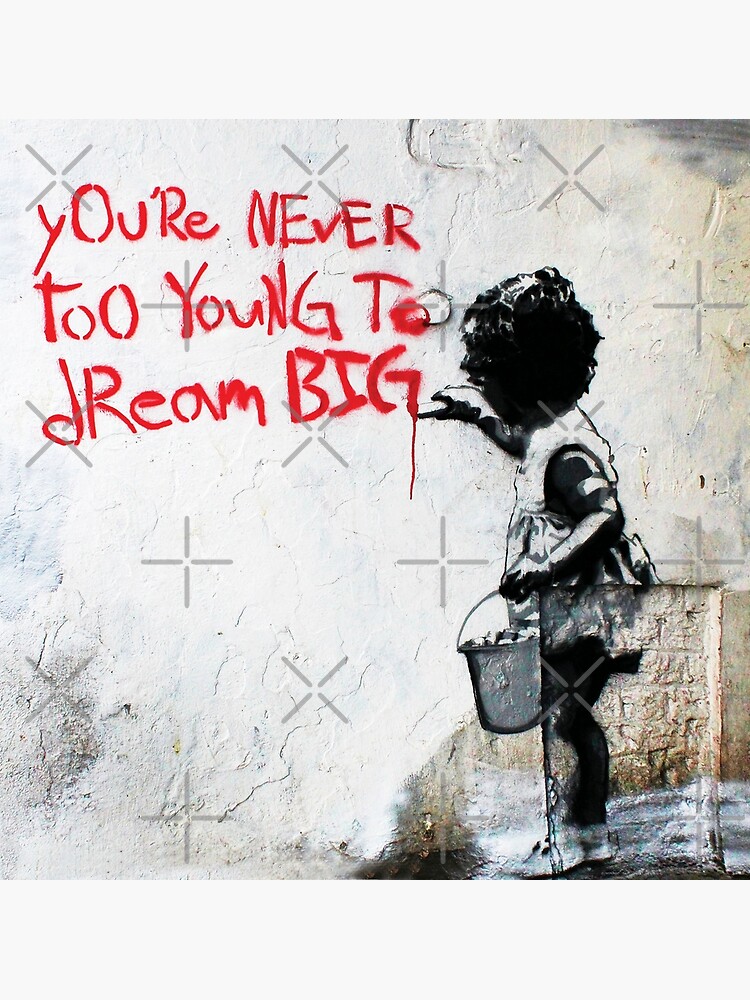The image depicts an aged, white-painted concrete wall, showing signs of wear and cracks. On the top left in red spray paint, the message "you're never too young to dream big" is written in a childlike, whimsical font with random capitalizations, such as a lowercase 'd' and an uppercase 'R' in "dream." Adjacent to this message on the right, there is a detailed graffiti illustration of a young child, viewed from the side but with their head turned away, showing only the back. This child, depicted in black outline, appears to be a young girl dressed in a simple outfit. She holds a pail in her left hand and extends her right hand as if she has just finished drawing the message with a piece of chalk. The child’s white shoes stand out against the backdrop. The wall’s surface also features crosses and signs of aging, contributing to an evocative street art tableau that merges playful innocence with an inspirational message.